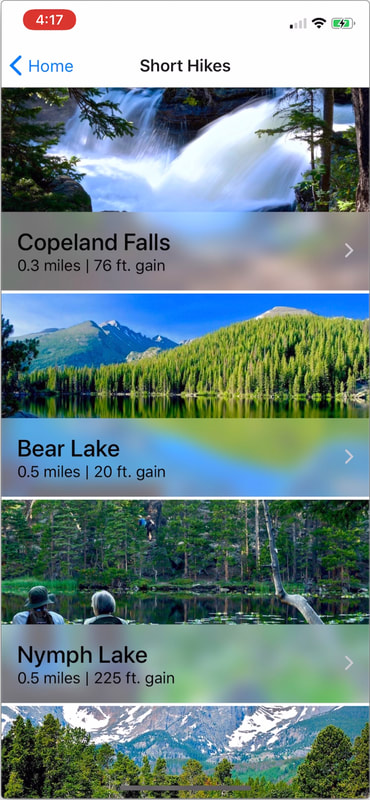This is a detailed screenshot of a phone displaying a hiking app interface. At the top, a red oblong-shaped box with a white border displays the number "417." The phone has 1 out of 4 signal bars, full Wi-Fi signal, and approximately 80% battery life remaining. Below this, a blue hyperlink with a left-pointing arrow labeled "Home" is present, next to black text reading "Short Hikes."

Under this header, an image depicts a picturesque waterfall surrounded by trees. In a gray information box at the bottom of the image, it states: "Copeland Falls, 0.3 miles, 76-foot gain."

Further down, another scene shows a mountain in the distance under a clear blue sky, with a forested hill and a serene lake in the foreground. The information box here reads: "Bear Lake, 0.5 miles, 20-foot gain."

Additionally, there is an image featuring a couple of people who appear to be either sitting in a boat or on the shore, presumably fishing. The water in this scene looks like a swamp. The label next to the image identifies it as "Mint Lake, 0.5 miles, 225-foot gain."

At the very bottom, a photo showcases a majestic glacier-filled mountain, framed by trees.